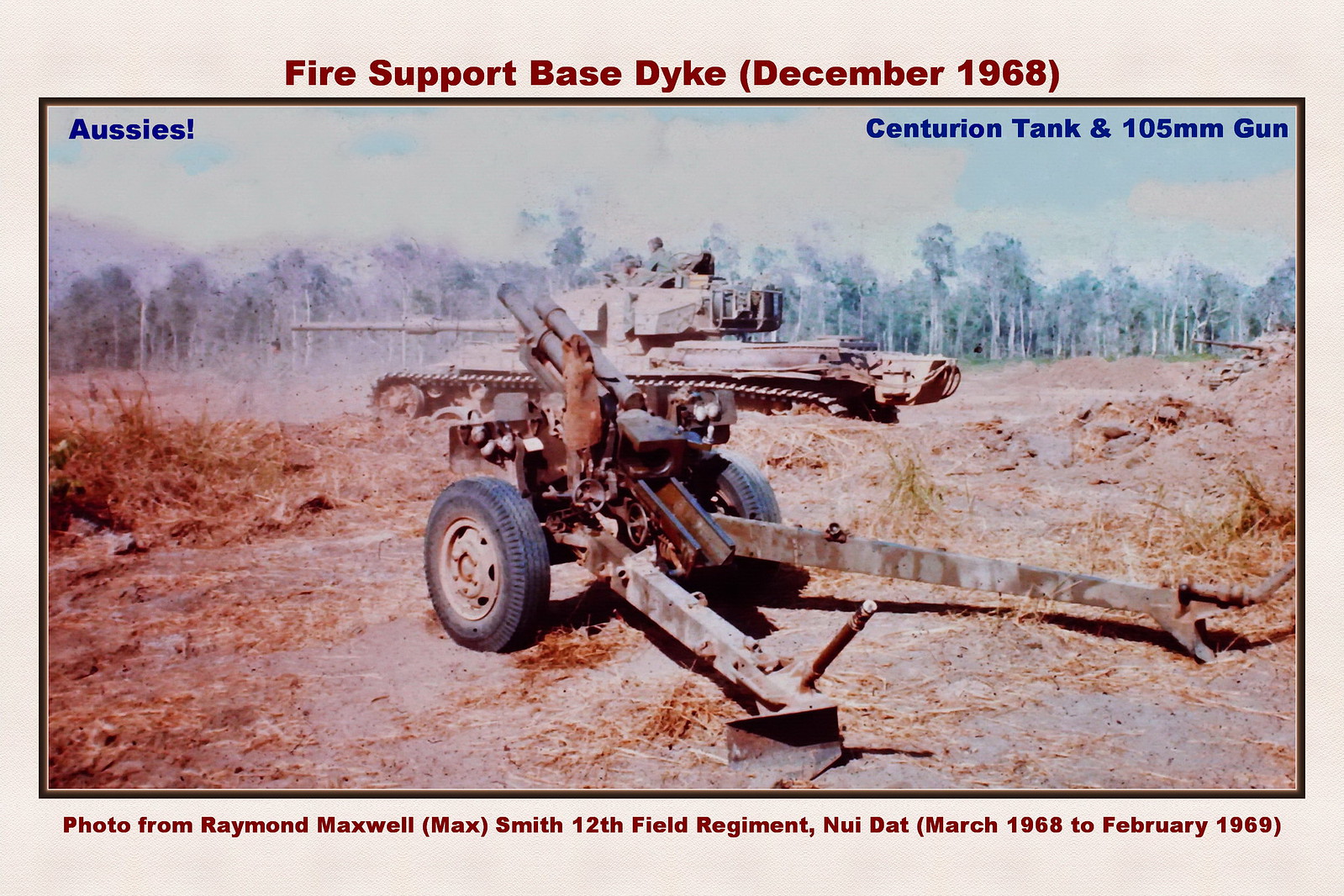The photograph captures a scene from the Vietnam War, surrounded by a thick tan border with a thinner dark brown line, creating a frame around the image. At the top of the tan border is red text reading "Fire Support Base Dyke (December 1968)," and at the bottom, it reads "Photo from Raymond Maxwell, Max Smith, 12th Field Regiment, Nui Dat, March 1968 to February 1969." Within the photograph, a large military cannon on wheels, capable of being hooked to a vehicle, dominates the foreground. The cannon points towards the top left corner, supported by its surrounding structure. Behind it stands a Centurion tank facing left, with its cannon aimed more towards the bottom left. The hazy background reveals a forest under a bright sky. In dark blue text at the top left of the image, "Aussies!" is prominently displayed. The ground around the equipment is brown grass and dirt, adding to the authentic war-time atmosphere.